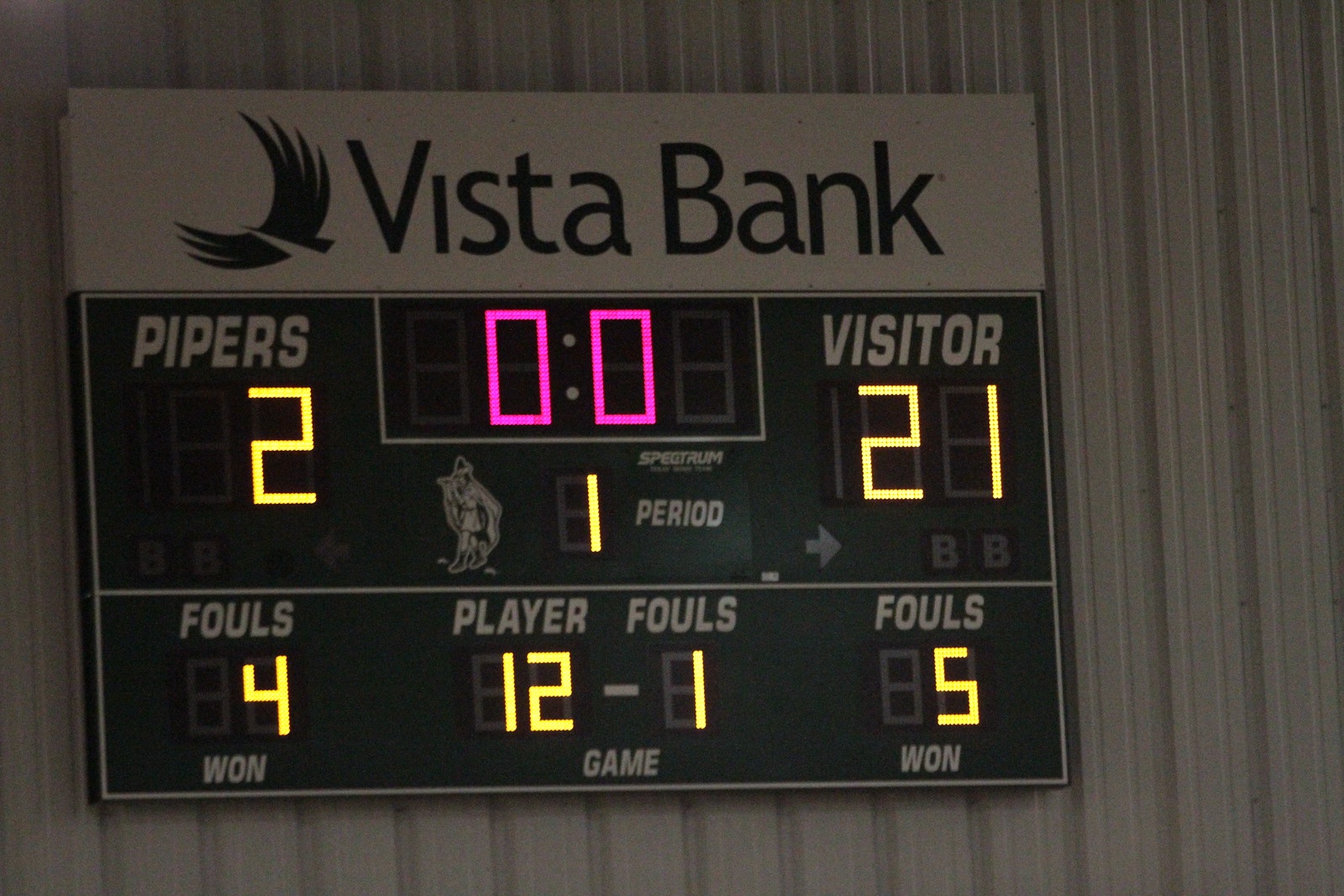This image depicts an older, black digital scoreboard mounted on a metal-framed wall, possibly located in a basketball gymnasium or a community center with brown, dark grey, and light grey partitions and vertical lines. The top of the scoreboard features a sponsor name, "Vista Bank," accompanied by a logo resembling an eagle with spread wings. The scoreboard's colored elements include a pink LED timer display showing double zeros, indicating no time left in the first period.

The home team, labeled as the Pipers, is trailing with a score of 2, while the visiting team is leading with 21 points. Both team names and their respective scores are displayed in yellow font. Foul counts are shown at the bottom corners, with the Pipers having four fouls and player 12 on their team marked with one foul, while the visitors have five fouls with one additional foul noted. The phrase "game" is also visible below the fouls section. Overall, the image captures the moment at the end of the first period where the home team is significantly behind.